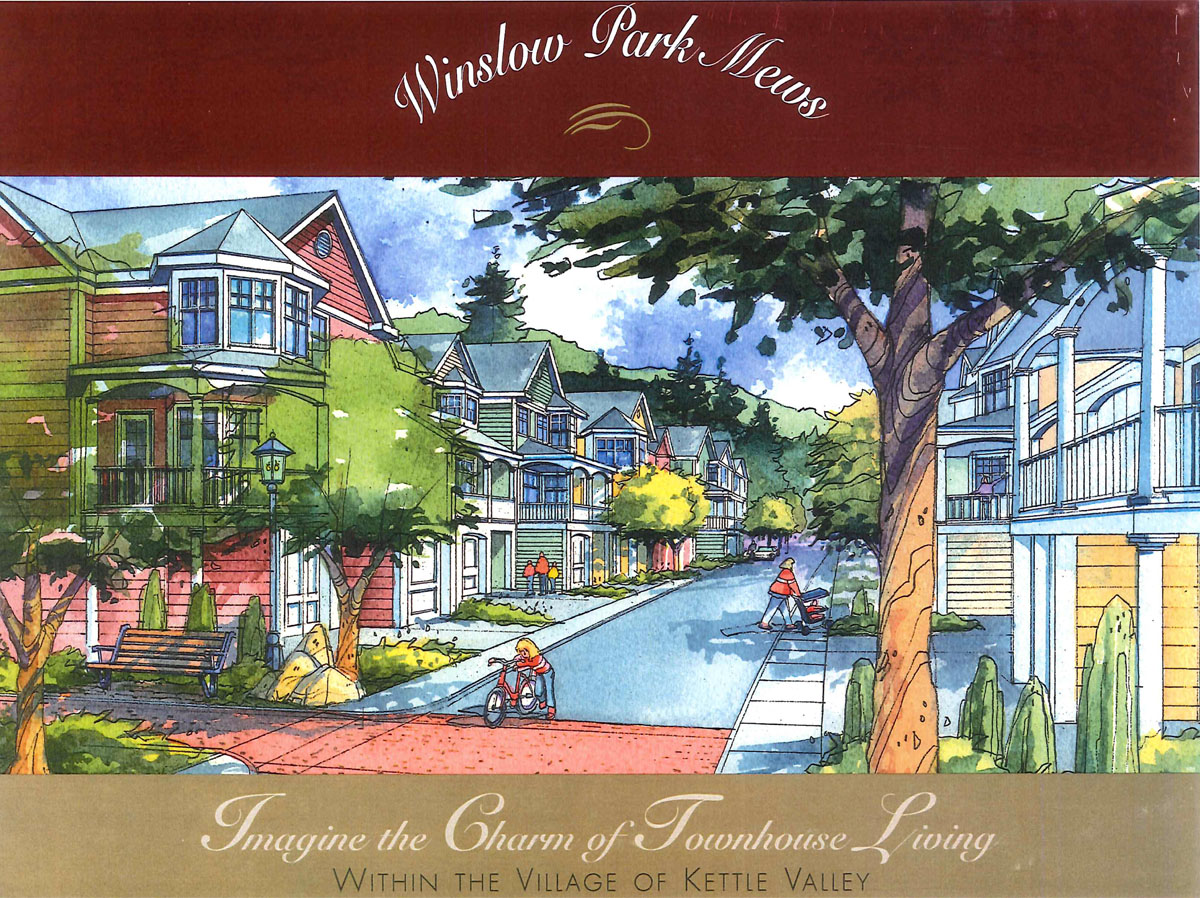The image is an advertisement placard that features a whimsical illustration of a picturesque neighborhood. At the very top, a maroon banner with elegant white cursive script reads "Winslow Park News," accompanied by a gold insignia logo. Below this banner is a colorful artist's depiction of a serene street scene. The street is a striking blue, along which a person is seen riding a bicycle and another pushing a stroller, creating a lively yet peaceful atmosphere.

Both sides of the street are lined with various two-story houses, many of which feature charming balcony structures and attached garages. These homes come in different shades, including red, green, and yellow, and are decorated with architectural details like pillars. The neighborhood is surrounded by numerous trees, under a clear blue sky with a backdrop of distant hills, emphasizing its lush and well-maintained environment.

At the very bottom of the image, a dark brown banner contains the phrase "Imagine the charm of townhouse living within the village of Kettle Valley" in white cursive script, inviting viewers to envision a life of quaint and desirable community living. This idyllic scene captures the essence of modern, comfortable townhouse living in a charming village setting.